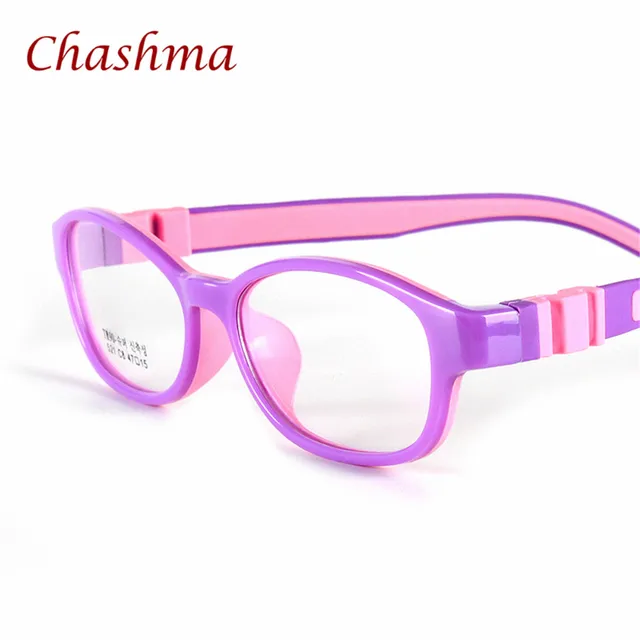The image features a pair of children's glasses prominently positioned in the center against a white background. The glasses have a striking design with an exterior frame in a vibrant purple color and a contrasting light pink interior, including pink nose pads and pink banding where the lenses meet the frames. The flexible arms of the glasses also show a mix of these colors, with the inner portions of the arms being light pink. There is detailed, unreadable text on the right lens, including some Asian characters. In the upper left corner of the image, there is the word "Chashma" or "Cheshire" in a rose-colored font. This well-lit, high-resolution photograph, likely intended for a sales website, showcases all the intricate details and dual-color design of the glasses.